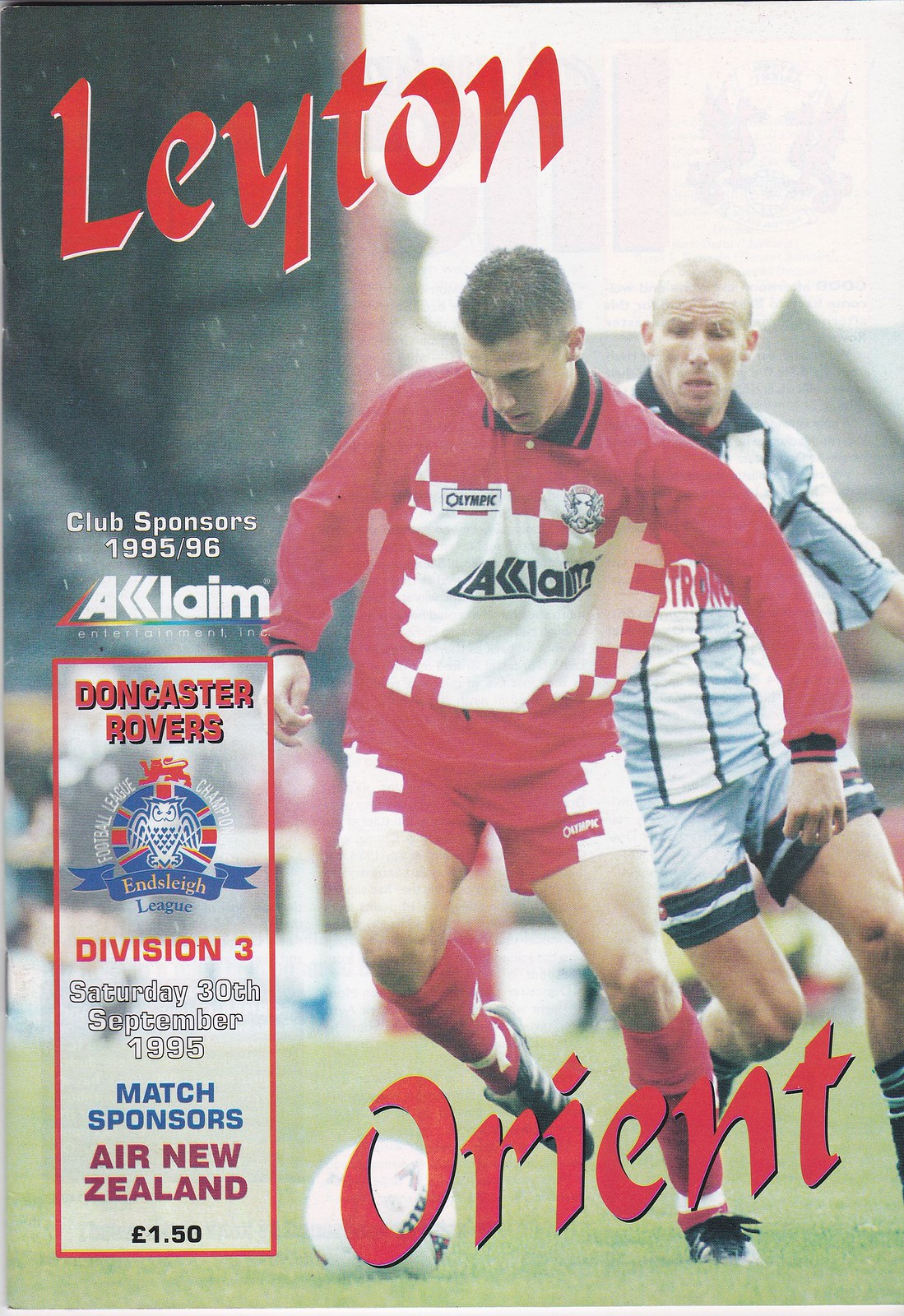This image serves as the cover photo for a football (soccer) program, specifically for a match between Leighton Orient and Doncaster Rovers. Dominating the scene are two players competing for the ball: the one in the foreground is dressed in a red and white long-sleeved jersey with a distinctive checkered pattern on the sides, paired with matching red and white shorts and socks, who appears poised to kick the ball. Behind him trails a player clad in a vertically striped jersey of blue, black, and white, accompanied by blue and black striped shorts and similarly colored socks, who seems to be challenging for possession.

Prominently displayed across the top of the program in bold red lettering is "Leighton," while "Orient" is similarly positioned at the bottom. On the left side, the text reads "Club Sponsors 1995-1996," featuring "Acclaim Entertainment." There's also a text box in the bottom left corner indicating "Doncaster Rovers," along with an emblem and the notation "Division 3." Further details highlight that this is a Saturday match, dated 30th September 1995, with "Air New Zealand" as the match sponsor. Also noted is that the program is priced at £1.50. Subtle elements like a visible section of the pitch and a glimpse of the crowd in the background add depth to the scene.